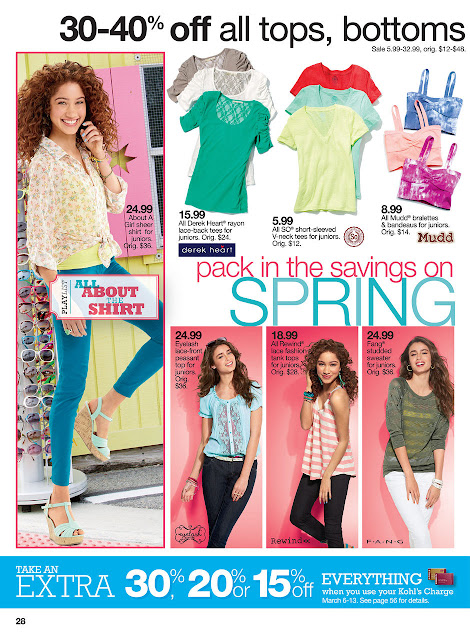**Detailed Caption:**

The image is a digital advertisement circular from Kohl's, resembling those weekly sales flyers typically found in Sunday newspapers. At the very top, the heading prominently displays "30 to 40% off" in bold black text, followed by "all tops, bottoms" in the same size font but not bolded. 

On the left side of the image, a teenage girl stands in front of a sunglass rack. She has long curly hair, is wearing skinny jeans, a floral top layered over a camisole, and wedge shoes. Text overlaying her image reads, "All about the shirt."

In the upper middle section of the circular, on the right side, there are images of three different types of tops stacked on each other. The first set of tops, priced at $15.99, are displayed to the left, next to a stack of v-neck t-shirts marked at $5.99 each in the middle. To the far right are three images of brassiere-style crop tops priced at $8.99 each.

The central text of the advertisement enthusiastically states, "Pack in the savings on spring." Below this, the circular continues to showcase a variety of young girl and teenage clothing options with more advertisements highlighting the available discounts and styles.